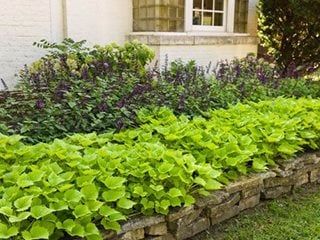In this daytime photograph, a serene garden scene is depicted with a stone retaining wall at the bottom, composed of silver and pale-toned stones. Above the wall, a lush assortment of green leafy bushes is showcased, varying in shades from lighter greens at the front to deeper greens towards the back. Nestled amidst these bushes is a white-painted house, partially visible with a glimpse of a white window complemented by shutters. The window glass reflects the surrounding greenery. Delicate bluish flowers appear to adorn the row of bushes at the back, adding a touch of color to the verdant landscape. Short, well-kept grass covers the foreground, completing this picturesque garden view.